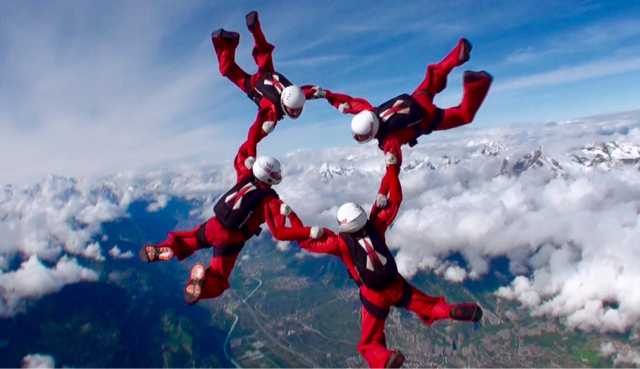In this thrilling horizontal image, skydivers are captured from above, likely from the plane they just exited. Below them stretches a vast expanse of the blue sky, interspersed with both puffy, marshmallow-like white clouds and soft, smoke-like gray clouds. Through these clouds, the earth is faintly visible, appearing green and brown with discernible roads winding below. The four skydivers, clad uniformly in striking red jumpsuits, form an interconnected circle by linking their arms. Each wears a white helmet and a black parachute backpack, detailed with a distinctive white stripe and a hint of red. Their legs are bent upwards at the knees, and they gaze intently at each other, enhancing the unity of their formation. Their footwear is coordinated, predominantly featuring black soles, with one diver sporting noticeable red soles. This perfectly arranged pose seems designed to capture a memorable moment against the dramatic backdrop of the sky and clouds.